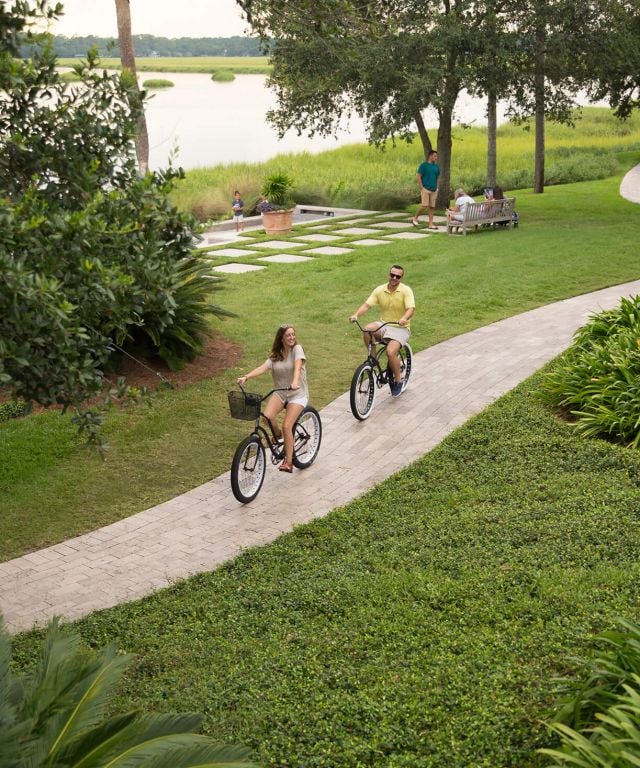This daytime photograph captures a charming summer scene in a lush, green park likely designed for both picnicking and leisurely enjoyment. The foreground features a stone brick bike path where a smiling woman—dressed in a gray shirt and white shorts—leads on a beach cruiser bicycle equipped with a black basket and wheels. Behind her, a man in a yellow polo shirt and gray shorts follows on a similar bicycle. The environment is enveloped in abundant greenery including manicured lawns, scattered bushes, and towering trees. 

To the side of the path, a bench is occupied by an older lady, a younger lady, and a child playing nearby, while a man stands close to them, possibly part of the group. The photograph also depicts a large potted bush on a concrete section, further adding to the sense of an intricately landscaped area. The scene extends towards a hazy sky above a body of water—likely a lake—buffered by a wide expanse of grass and marshy areas. The overall hazy atmosphere and details of the clothing and bikes give the image a nostalgic touch, as if the moment captured could be a modern-day reimagining of a setting from decades past.